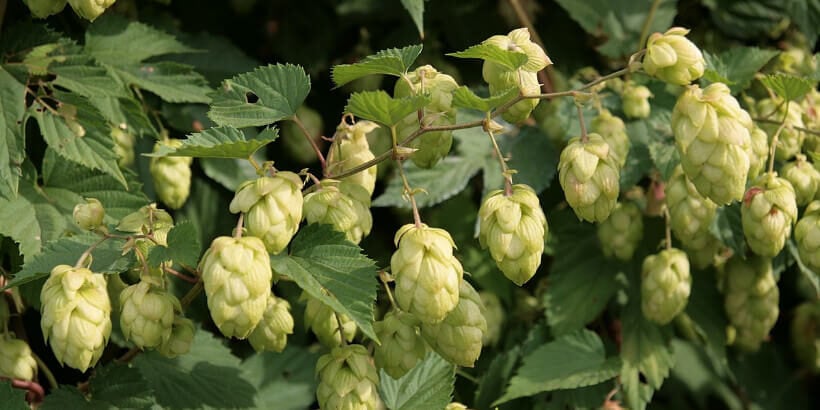The image captures a dense, horizontal shot dominated by leafy vines with closely packed, unopened buds. The scene, seemingly positioned outdoors in a brightly lit setting, highlights the rich textures and vitality of the green foliage. Despite the buds not revealing whether they're flowers or vegetables, their tightly clustered forms add a sense of anticipation. The colors range from vibrant greens to hints of yellow, brown, and occasional black and tan hues, suggesting a natural, earthy environment. Centered within the frame, the main plant's detailed portrayal suggests a setting akin to a hops farm, emphasizing the agricultural context.